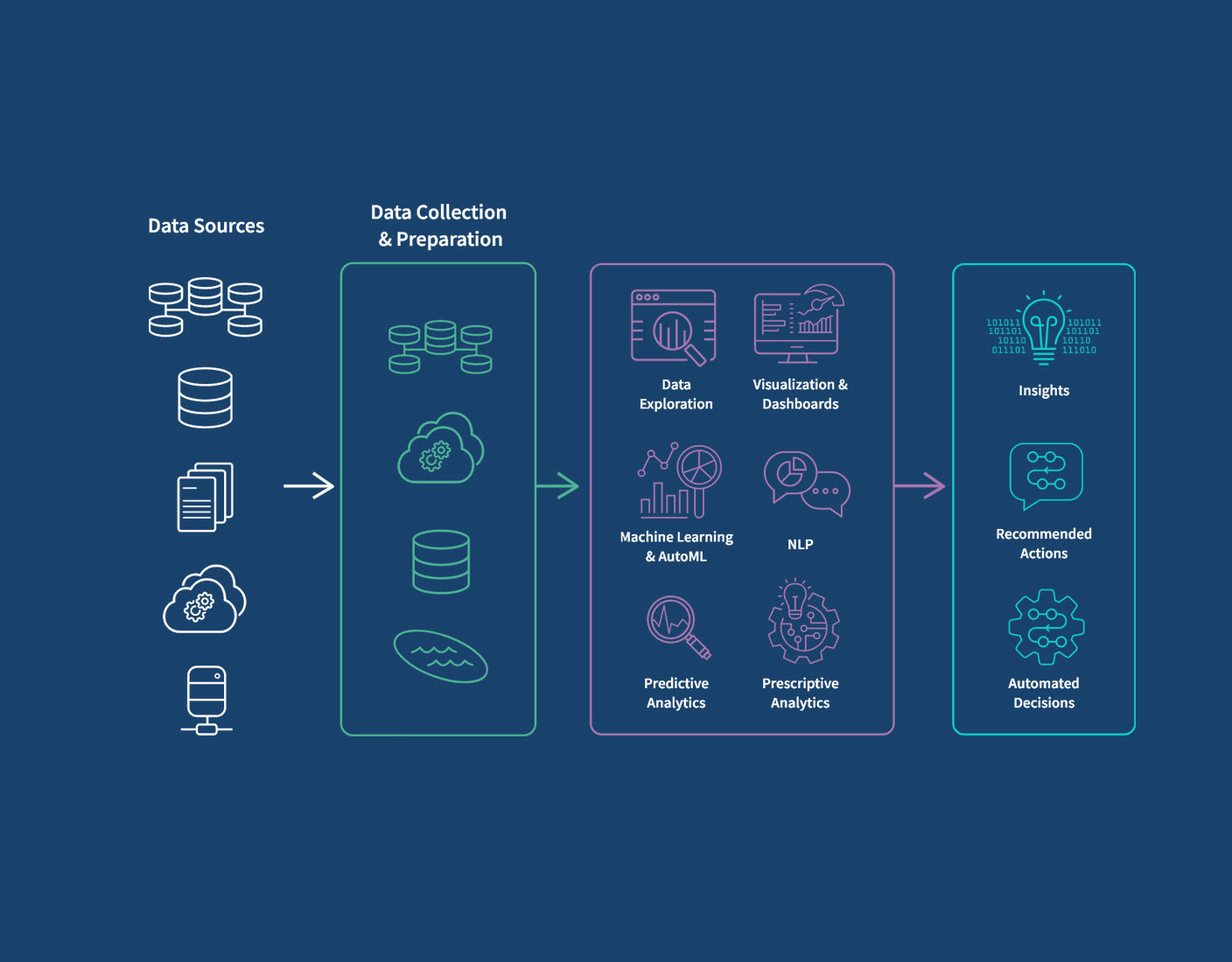The image depicts an informational diagram against a dark blue background, structured into five columns with directional white arrows guiding the flow from left to right, through a series of phases and processes. On the far left, a white-bracketed section labeled "Data Sources" features icons such as interconnected stacks of coins, single stacks of coins, sheets of paper, clouds with gears, and a small square object. Proceeding rightward, a light green arrow points to the next column, "Data Collection and Preparation," which encapsulates the same type of icons, this time framed in a light green border. Continuing along, a purple arrow leads to the third column, bordered in purple and titled "Data Exploration, Visualization and Dashboards, Machine Learning and AutoML, NLP, Predictive Analytics, and Prescriptive Analytics," also depicted in purple graphics. Finally, a green arrow directs towards the fourth section marked by a green border, which emphasizes "Insights, Recommended Actions, and Automated Decisions." This detailed diagram effectively visualizes the comprehensive process from raw data collection to actionable insights and decisions.